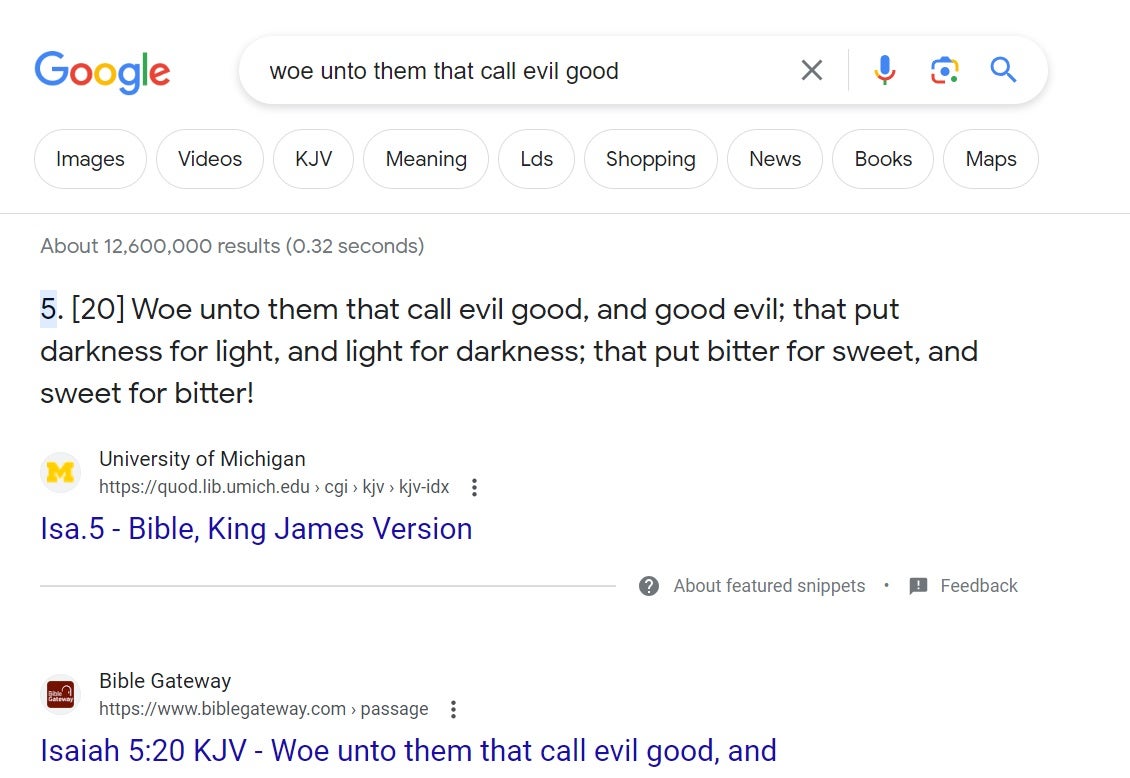This image captures a Google search results page against a white background with predominantly black text. In the upper left corner, the iconic Google logo is displayed in its distinctive colorful letters. To the logo's right, a search bar shows the input query: "woe unto them that call evil good."

The first search result is highlighted, displaying the text: "Woe unto them that call evil good and good evil, that put darkness for light and light for darkness, that put bitter for sweet and sweet for bitter." Below this text, a link to the University of Michigan’s website is provided, followed by a description indicating that this is a passage from the Bible, specifically Isaiah 5:20 in the King James Version (KJV).

The second result lists another source, Bible Gateway, with a corresponding web address: www.biblegateway.com/passage/Isaiah 5:20 KJV. This result also references Isaiah 5:20 and again partially repeats the verse: "Woe unto them that call evil good and…" before being truncated.

Overall, the image presents Google search results for a significant Biblical quote from Isaiah 5:20 in the King James Version, showing different sources where this passage can be found and read in full.